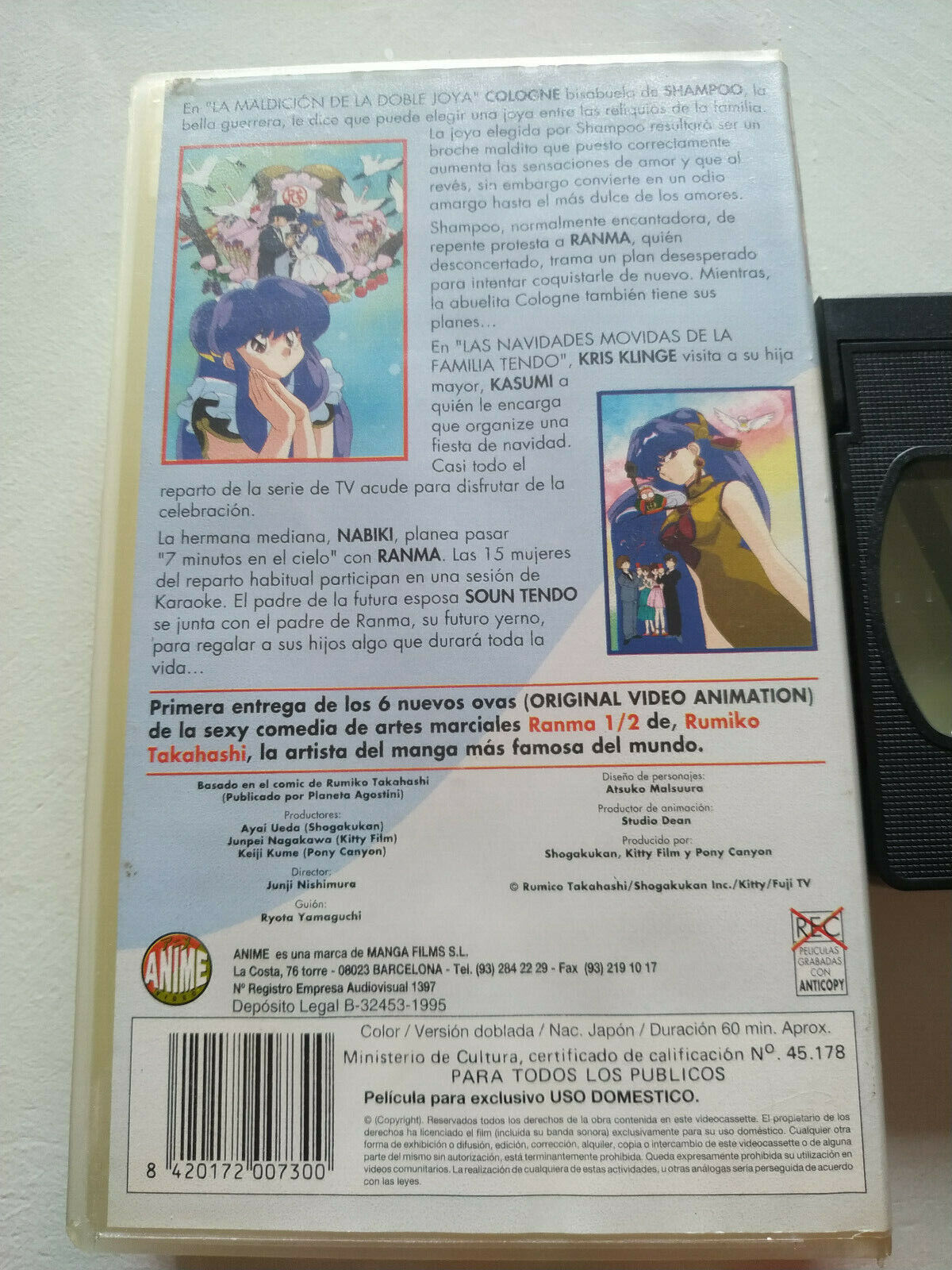This image displays the back side of a VHS tape or potentially a DVD of an anime series or movie, featuring text predominantly in Spanish. The background is predominantly bluish-white, adding a crisp contrast that makes the text easy to read. In the upper left corner, there's a photo of an anime character with blue hair, and in the lower right corner, another image depicts a girl with blue hair in an olive-colored sleeveless dress, both seemingly looking towards the camera. Below these images, additional text references characters such as Ranma, Nabiki, Kasumi, Cologne, and Kris Klinge. There is an anime logo located in the lower left corner of the cover. At the very bottom, a barcode is visible alongside information about the tape, such as its color version, duration, and presumably other relevant details, all written in Spanish.